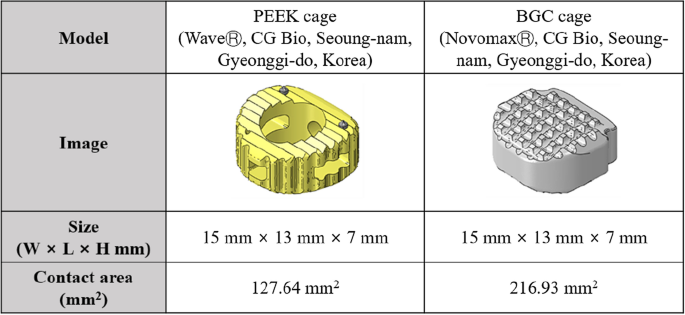The diagram from Seongriya presents a comparative model of two types of cages: the gold-colored 'Peak Cage' and the silver-colored 'BGC Cage.' This detailed chart consists of four rows and three columns, with the leftmost column shaded light gray and the remaining columns in white. The rows are titled 'Model,' 'Image,' 'Size,' and 'Contact Area.' The diagram displays the measurements of both cages, each being 15 millimeters by 13 millimeters by 7 millimeters, along with additional dimensions of 127.64 millimeters and 216.93 millimeters. The 'Peak Cage' is distinguished by its unique yellow/gold piece that appears to be hollow, while the 'BGC Cage' is solid, providing a larger contact area. The design of the cages includes features reminiscent of a claw hammer without a handle and a set of tooth-like structures. The chart also references WAVE-R and NOVOMAX-R by CG-Bio, based in Sungnam, Gyeonggi-do, Korea.